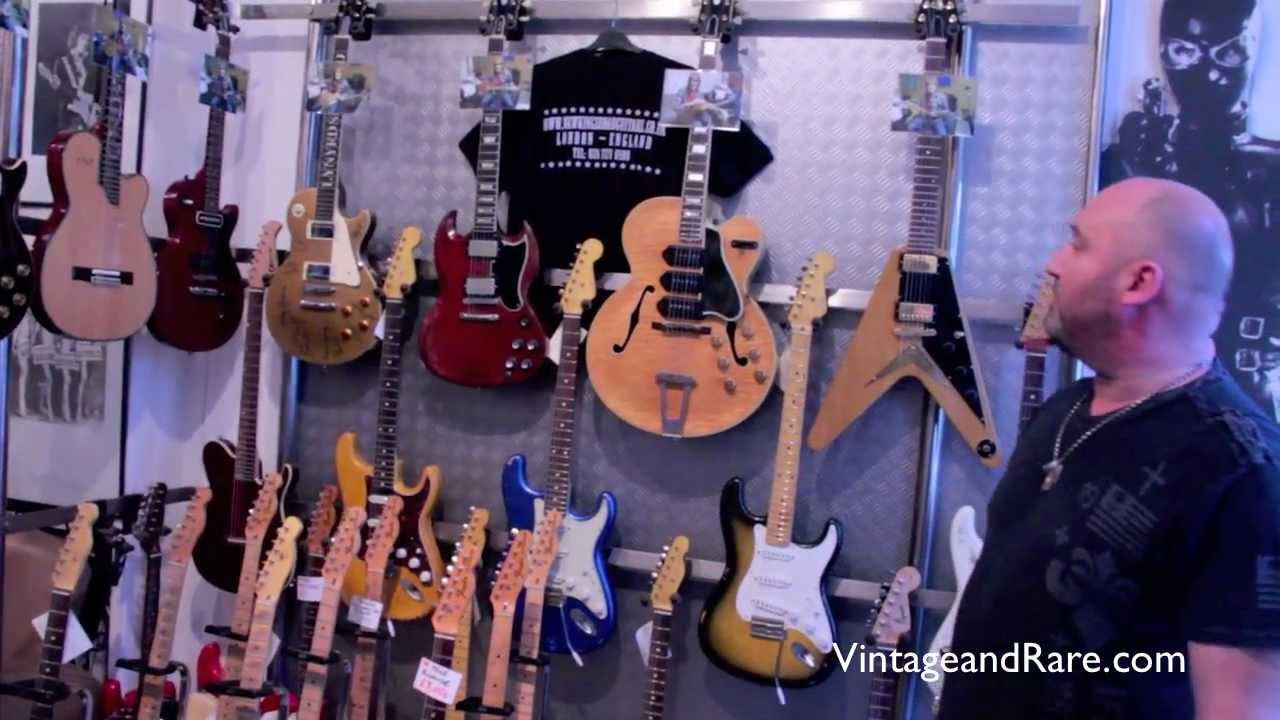In this detailed image of a guitar store, an extensive collection of electric guitars is displayed on a metallic gray wall. The guitars, ranging in colors from light brown to darker red, and including a distinctive blue one, are meticulously arranged in upright rows with their necks pointing upward. Some guitars are mounted directly on the wall, while others are standing on the floor with the help of stands. Each guitar features a small picture near the neck, likely depicting the musicians who played them. Prominent guitar brands such as Gibson, Les Paul, Fender, and unique shapes like Flying Vs are visible. On the lower right, the watermark "Vintage and Rare.com" is displayed in white font.

A bald man stands on the right side of the image, gazing up at the guitars. He has a fair complexion and wears a black, short-sleeved T-shirt adorned with various gray graphics, including a cross and an American flag. Around his neck is a metal necklace with a pendant that resembles the head of a horse. A poster of a figure in a black mask and leather attire, pointing a gun, is visible on the upper right side of the wall, adding a touch of intrigue to the scene.